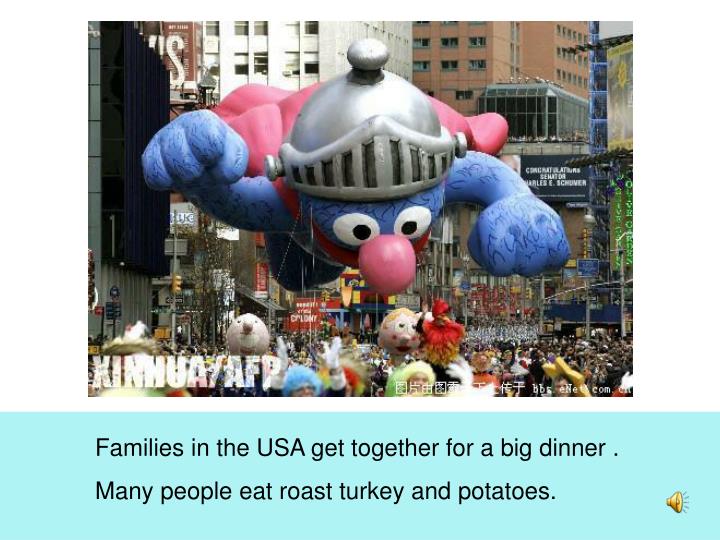The image captures a bustling city scene during the Macy's Thanksgiving Day Parade. Dominating the mid-ground is a gigantic float balloon of Super Grover from Sesame Street, characterized by his blue body, wide eyes with black pupils, signature big pink nose, silver knight-like helmet, and flowing red cape. The backdrop features towering buildings, at least ten stories high, with a white building in the foreground and a brown one further back. Below the floating Super Grover, a crowd of hundreds of people, some holding down the balloon's ropes and others dressed in various cartoon character costumes, fills the street, highlighting the grand scale of the parade. The image conveys the festive atmosphere of this iconic American event, with families gathered to celebrate amidst the vibrant cityscape.